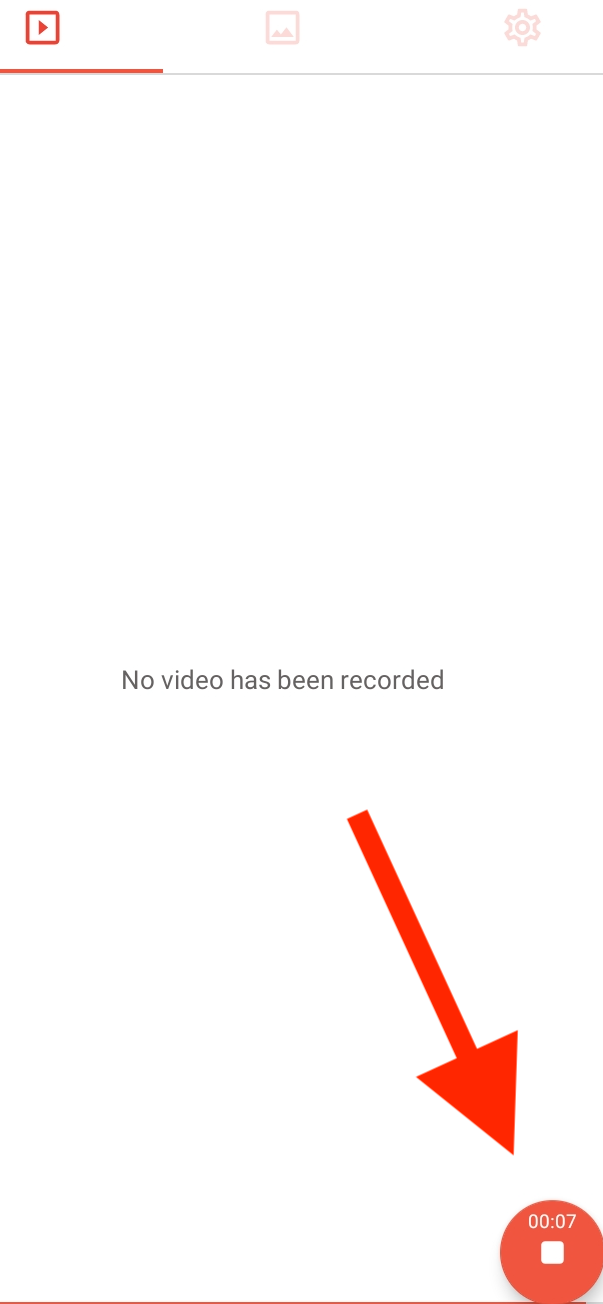The image depicts a predominantly white webpage designed to resemble an app interface. At the top, there is a navigation bar featuring three buttons. 

On the left, a prominent red square encloses a white play icon, indicating the selected video mode. This selection is emphasized by a red underline just beneath the button. 

Next to it, a similarly styled square with an icon of mountains signifies the photograph mode. While also red, this button is lighter in color, showing it is not the current selection. 

Furthest to the right on the top bar is a gear icon, representing the settings. This button is a pale, muted red, further indicating it is not actively selected.

Centered in the main portion of the screen, a message reads, "No video has been recorded." 

Below this message, a large red arrow points towards the bottom right corner of the screen, directing attention to a stop button. This button is displayed as a red circle with a white square in its center and shows a timer at seven seconds.

The bottom of the page is marked by a solid red line, signifying the end of the webpage.